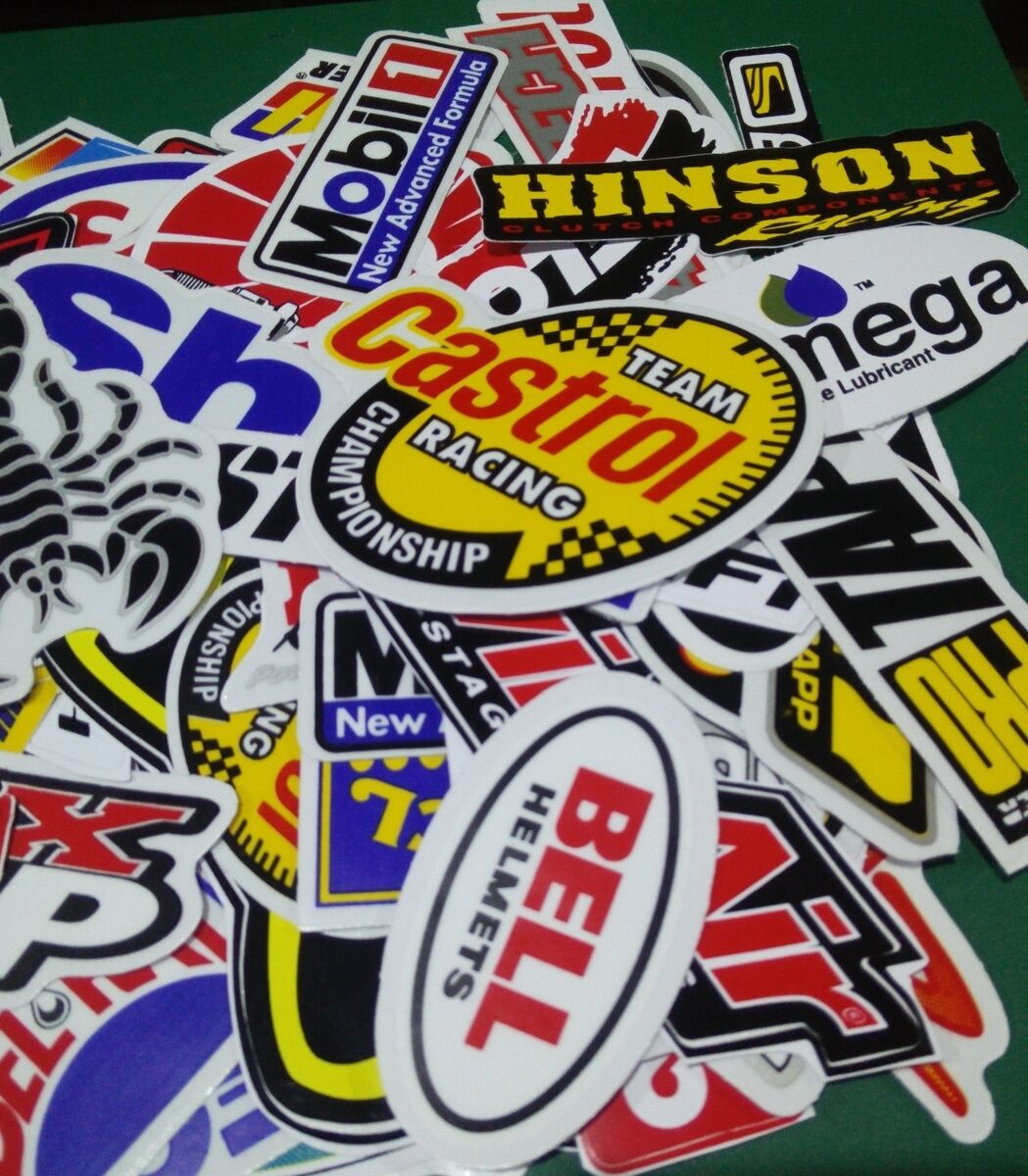This photograph captures a chaotic pile of adhesive stickers or decals, likely related to racing or automotive themes, scattered on a dark green background reminiscent of pool table felt. Prominently, there is a red, white, and blue Mobil 1 sticker labeled "New Advanced Formula," and a bold yellow sticker with "Hinson" in black letters. Another notable decal features a bright yellow circular design with the words "Team Castrol Racing Championship" in various colors and fonts, including red and white. An oval white sticker with red "Bell" text and "Helmets" in black sits at the bottom. Partially visible is another white oval sticker with blue and green teardrop shapes and the word "M-E-G-A," followed by "Lubricant." Additional partial stickers with varied icons and text add to the densely layered cluster, hinting at their automotive nature but remaining obscured by the overlapping arrangement.